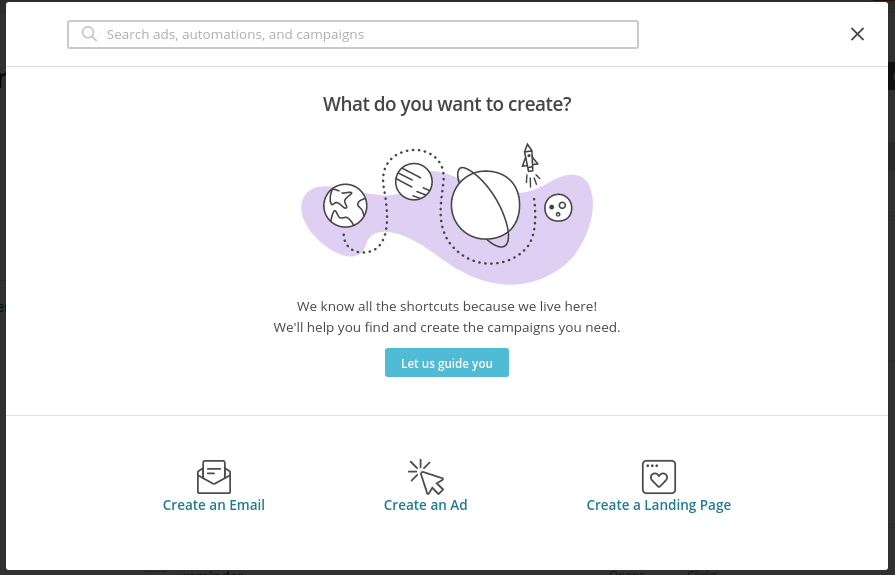The image has a white background with a black border. At the top, there is a search bar with the options: "Search," "Ads," "Automations," and "Campaigns." To the upper right corner of the search bar, there is an 'X' icon for closing the search. Below the search bar, in black text, it reads, "What do you want to create?"

Below the text, there is a series of colorful illustrations, outlined in black. These include:
- A purple blotch
- A depiction of Earth
- Another planet resembling either Neptune or Saturn, indicated by its rings
- A rocket
- A moon-like object

A dotted line starts from Earth, curves around the other planet, and then under the depiction of Saturn, finally moving upwards between Saturn and the moon object. Accompanying this graphic, there is a tagline in black font: "We know all the shortcuts because we live here. We’ll help you find and create the campaigns you need."

Further down, there is a turquoise button with white text saying, "Let us guide you." Below this button, there are three options depicted in black with small illustrations:
1. "Create an email" – illustrated with an envelope containing a letter.
2. "Create an ad" – accompanied by a cursor arrow that appears to be clicking.
3. "Create a landing page" – shown with a square website page icon containing a heart.

The overall design uses a primarily black font with some teal coloring for emphasis. The image lacks any specific indication of its source or website information.